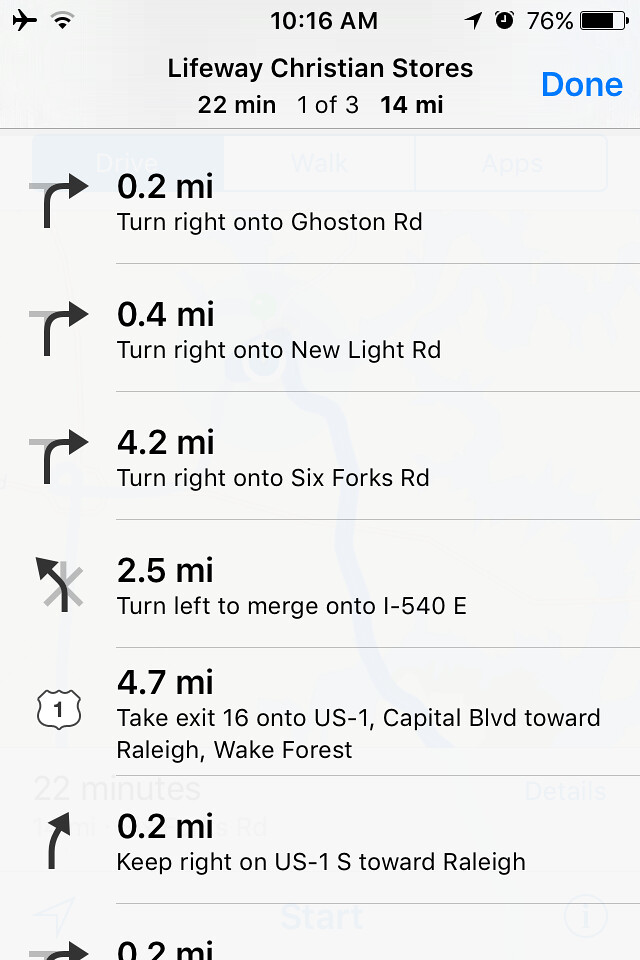The image is a screenshot of an iPhone displaying navigation directions to Lifeway Christian Stores, which is 22 minutes away and 14 miles distant. At the top of the screen, the status icons show the phone is in airplane mode, connected to Wi-Fi, and has 76% battery life with an alarm set. The current time is 10:16 a.m. The background of the screen is a light gray, with a route map faintly visible behind the directions. The step-by-step directions are as follows: In 0.2 miles, turn right onto Ghoston Road; 0.4 miles, turn right onto New Light Road; 4.2 miles, turn right onto Six Forks Road; 2.5 miles, turn left to merge onto I-540 East; 4.7 miles, take exit 16 onto US-1 Capitol Boulevard towards Raleigh and Wake Forest; and in 0.2 miles, keep right onto US-1 South towards Raleigh.